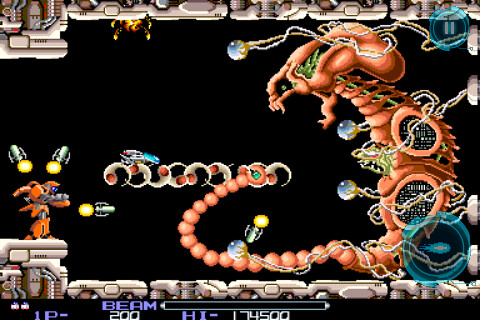In this gripping video game scene, the foreground is dominated by a colossal, menacing monster set against a stark black background. The beast features a grotesque, bladder-like structure at its top, adorned with several small, white pipe-like protrusions and greenish interior details. Its spine is reminiscent of curling, razor-sharp edges, while two spherical appendages dangle ominously below. The monster's tail, comprised of progressively smaller brown bead-like segments, trails off into the darkness.

Above this fearsome creature, the backdrop is dotted with numerous tiny, white, pipe-like formations. Adding a sense of scale and urgency, a small, brownish, multi-legged creature scurries nearby. Perched on a ledge to the right, a dog-shaped character, also brown in color, takes aim and fires relentlessly at the towering adversary, striving to vanquish the formidable foe.